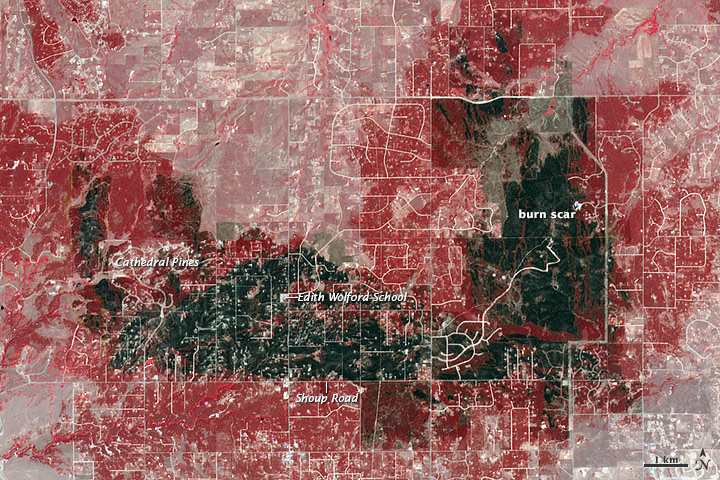This satellite image showcases a map overlaid with detailed information about an area ravaged by wildfires. The predominant feature is a large, irregular black area labeled "burn scar" in white letters, encompassing around 20-25% of the map, primarily on the right side and extending towards the lower middle and parts of the left side. The map displays roads and significant locations in white, against a red background indicating varying levels of fire intensity, with deeper red areas suggesting more severe burning. Notable landmarks include Edith Wolford School, marked with an arrow pointing to a small square on the map, and Cathedral Pines, similarly marked. Shoop Road is also identified as a small black square. The edges of the map have a lighter, cloudy white coloration, possibly representing cloud cover. A distance indicator at the bottom right corner notes "one kilometer," providing a sense of scale. This detailed map underscores the extensive damage wrought by the wildfires, highlighting critical infrastructures within the affected area.